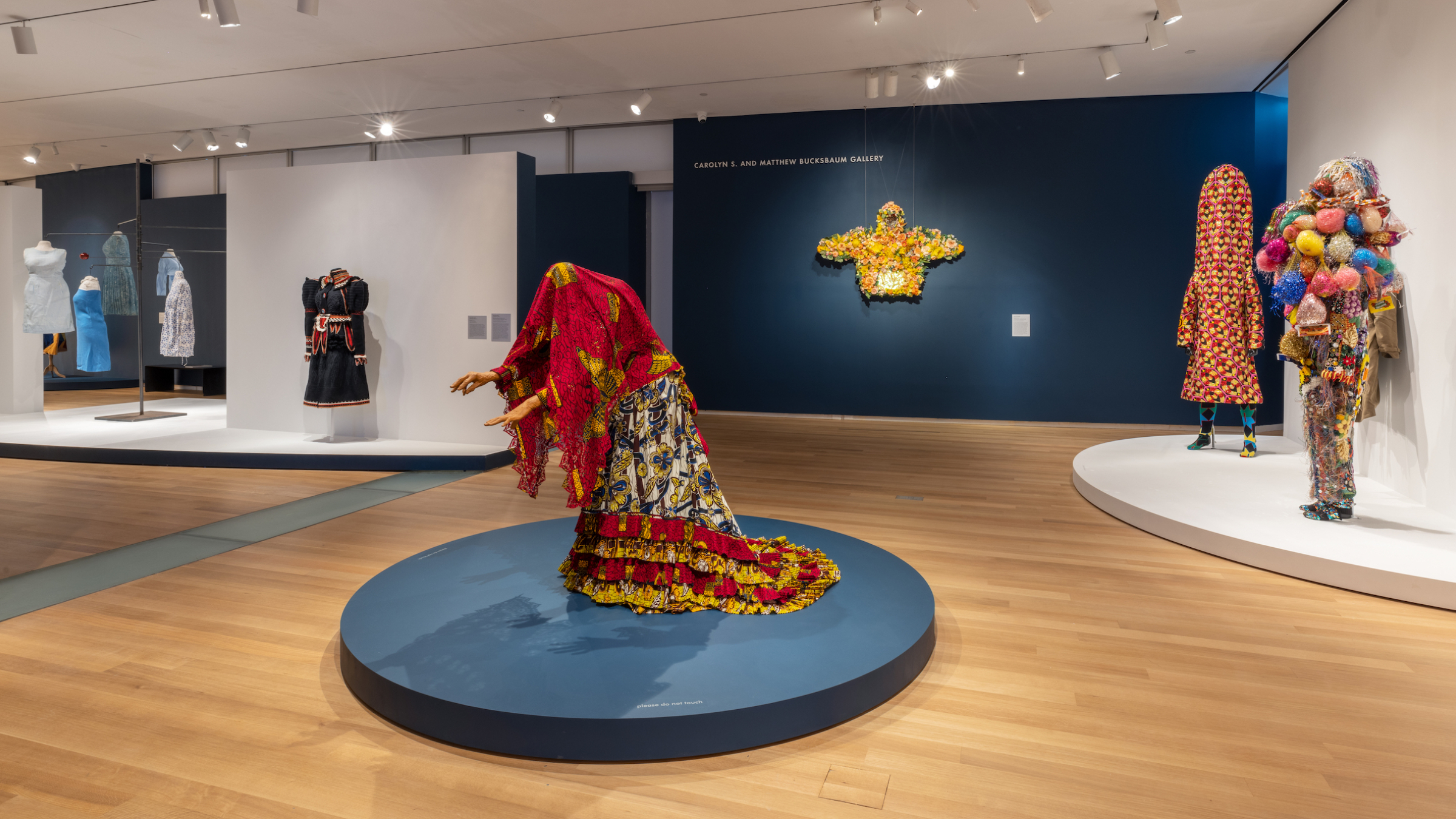The photograph depicts an exhibit from the Garmenting Costume as Contemporary Art collection at the Stephen Friedman Gallery in London, presenting a sophisticated and modern display of fashion pieces. The room features a striking interior with various focal points and platforms. Central to the exhibit is a round, blue circular stage showcasing a headless mannequin adorned in a long, colorful skirt with reds and yellows that flares out behind it. The mannequin is covered by a scarf that drapes over the entire body, extending into a red fabric hood.

To the left, a white wall and a free-standing white wall supported by a small stage are dressed with a series of elegant dresses, some positioned behind glass, while others stand freely showcased on platforms. Opposite this, a semi-circle white platform emerges from a blue wall, displaying two avant-garde costume designs: one featuring a mannequin entirely enveloped in a multi-digital print garment, and another festooned with an array of balloons, creating a futuristic aesthetic.

On the far back wall, a prominent golden hooded jacket hangs against a deep blue background, adding a touch of luxury and grandeur to the ensemble. This landscape-oriented, color photograph impeccably captures the essence of Photographic Representationalism Realism, emphasizing the artistry and contemporary flair of high fashion in a museum-like setting.